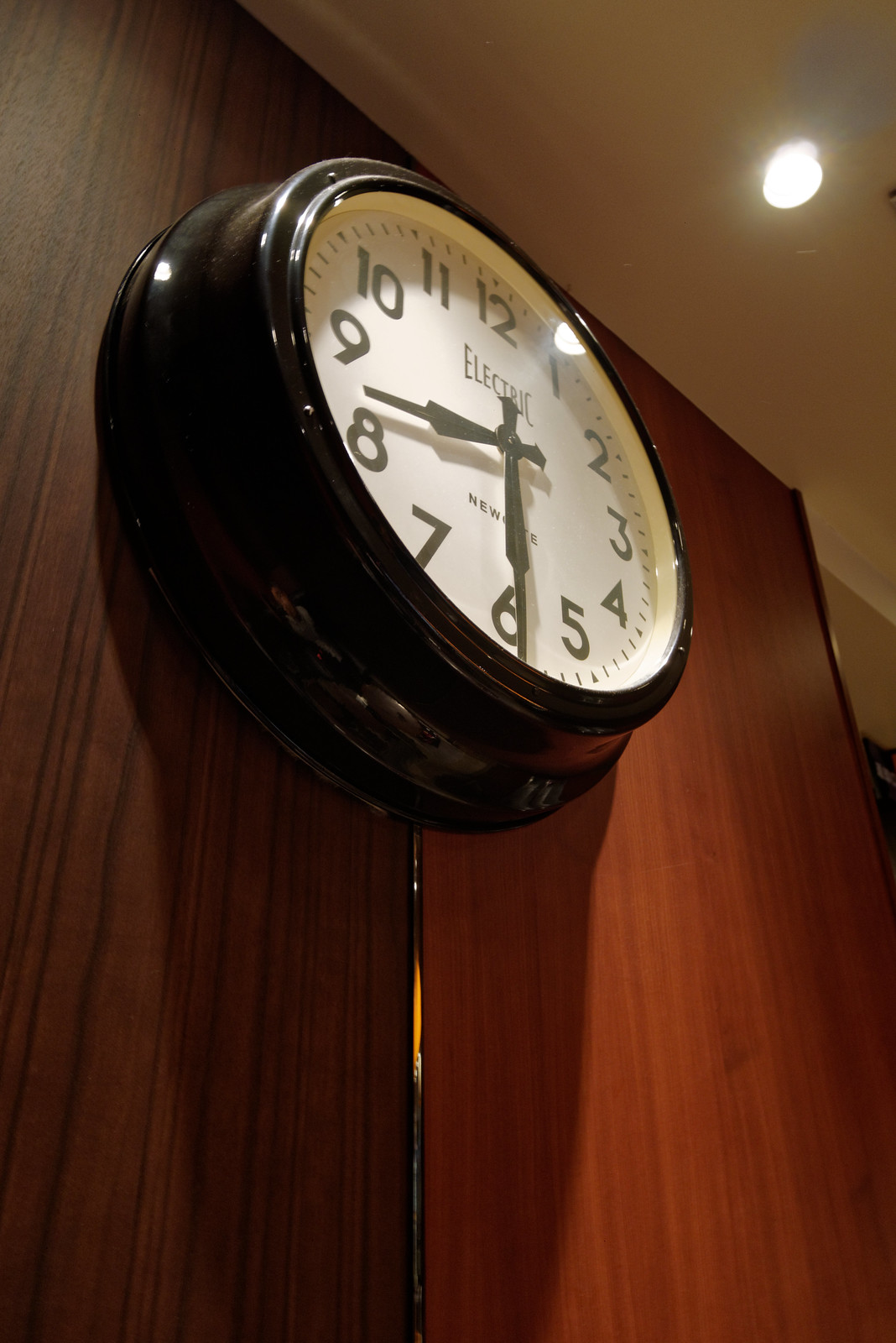The image features a classic wall clock with a white face, prominently displaying the brand name "Electric Newark" in bold black letters. The clock face is adorned with black numerals ranging from 1 to 12, and it has matching black hour and minute hands indicating the time as 8:29. Encased in a black border, the clock is mounted on a section of dark, split wood paneling, which suggests the presence of two hinged doors. Through the narrow gap between the panels, a faintly lit background is visible, hinting at an illuminated space behind the clock. Overhead track lighting casts a focused beam onto both the clock and the camera, accentuating the details against a white, unadorned ceiling.